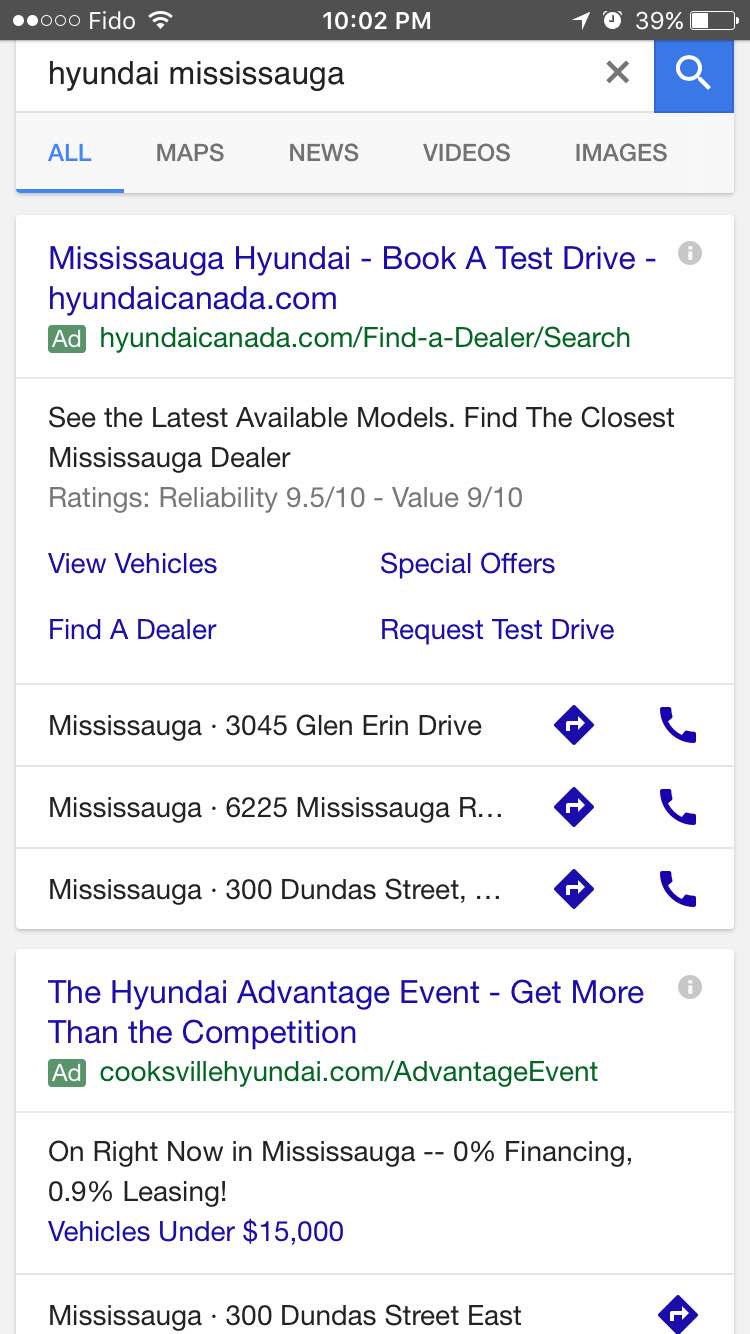**Descriptive Caption:**

The vertical rectangular image appears to be a screenshot, likely from a mobile device, detailing a Google search result for "Hyundai Mississauga." 

- **Header Section:**
  - The top features a horizontal black bar containing status icons:
    - On the left, two out of five circles are filled with white dots.
    - Centered is the time displayed as 10:02 PM.
    - On the right, the battery icon indicates 39% charge, nearly half filled with white.
- **Search Box:**
  - Beneath the black bar is a search box with the queried text "Hyundai Mississauga" in black font.
  - The right end of the search box contains a black 'X' and a vertical blue rectangle with a white magnifying glass icon.
- **Navigation Tabs:**
  - Following the search box, navigation tabs are displayed in all caps:
    - The first tab, "ALL," is highlighted in turquoise with a horizontal turquoise line underneath.
    - Other tabs: "Maps," "News," "Videos," and "Images," are in black font.
- **Search Results:**
  - The primary search result is an advertisement:
    - **Headline**: "Mississauga Hyundai, book a test drive" in a bluish-purple font, linking to HyundaiCanada.com.
    - **Ad Indicator:** A green square box labeled "Ad" in white.
    - **Description:** In green font, "HyundaiCanada.com/find a dealer/search"
    - **Details:** Black font - "See the latest available models, find the closest Mississauga dealer."
    - **Ratings:** In light black font - "Ratings: Reliability 9.5/10, Value 9/10."
    - **Call-to-Action:** In bluish-purple font - "View vehicles."
  - Further sections:
    - **Dealer Listings:**
      - In the center section, dealer addresses listed start with "Mississauga":
        - "3045 Glen Aaron Drive" followed by icons: a blue diamond with an arrow pointing up/right and a blue telephone receiver.
        - "6225 Mississauga" (cut off with same icons presumably).
        - "300 Dundas Street" with the same icons.
    - **Additional Ad:**
      - "The Hyundai Advantage event - Get more than the competition" followed by a green ad box.
      - Green font: "cooksvillehyundai.com/advantage event"
      - Black font: "On right now in Mississauga, 0% financing, 0.9% leasing."
      - Bluish-purple font - "Vehicles under $15,000."
      - Address: "Mississauga 300 Dundas Street East."